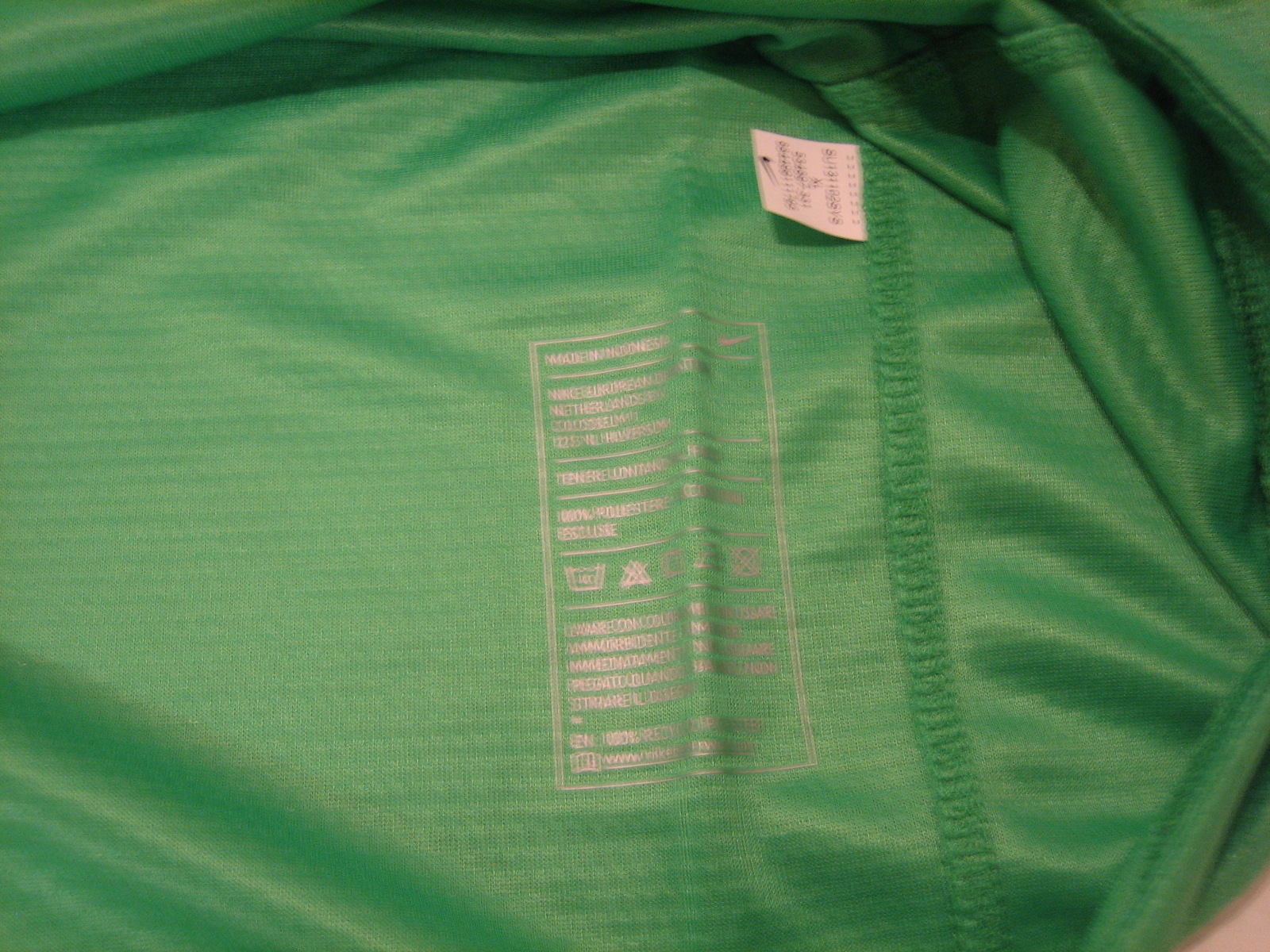A vibrant green shirt is displayed prominently. The shirt features intricate green stitching along the seams, enhancing its polished look. A small white tag is sewn into the inside neck, providing essential information. Additionally, a silver-toned tag, likely detailing laundry instructions, is affixed as well. The shirt exudes quality and attention to detail.